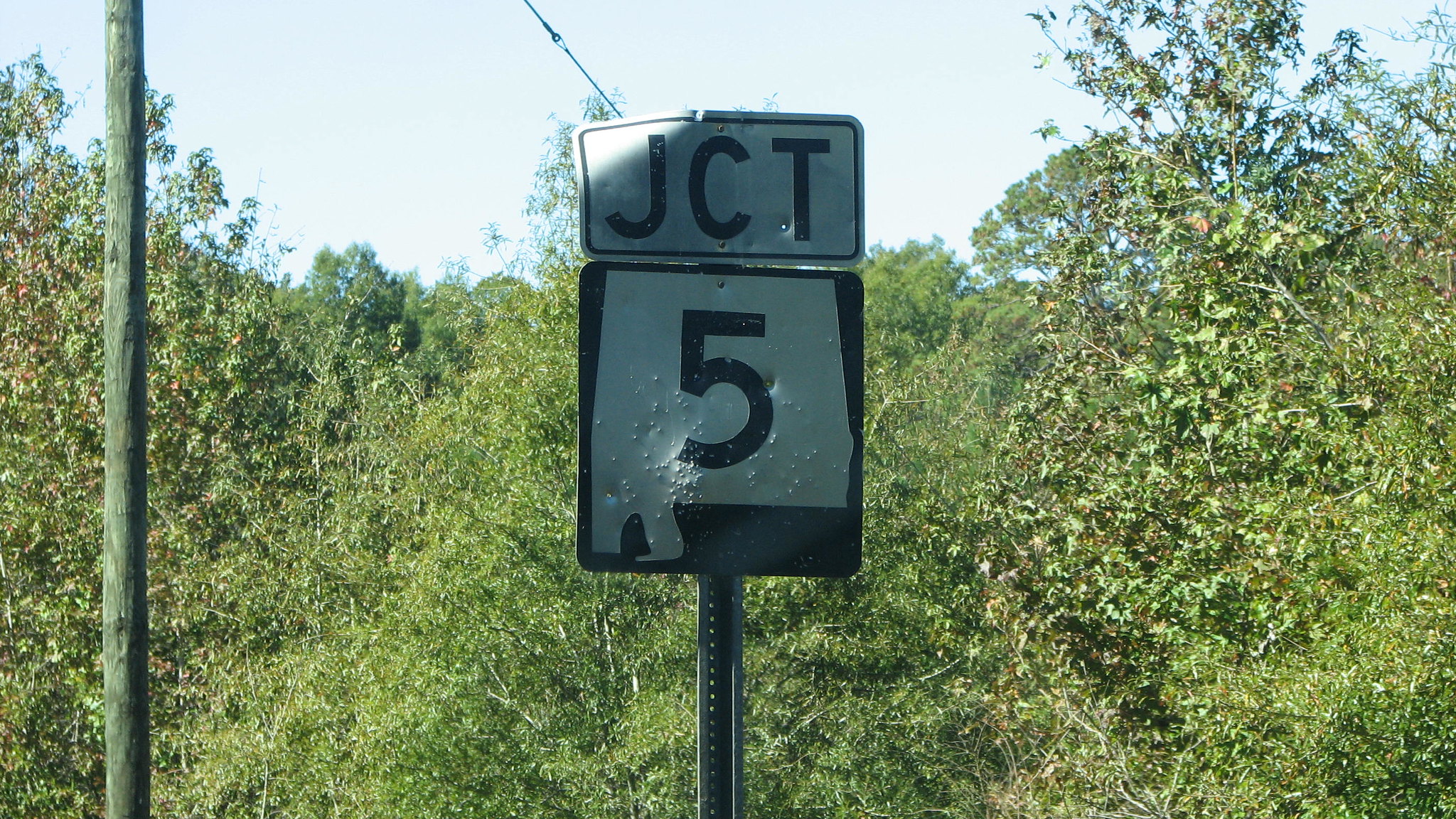This photograph, taken in a horizontal mode, captures a close-up of a weathered and damaged road sign mounted on a silver pole with numerous wind-resistant holes. The scene is bathed in sunlight, highlighting the details of the sign and its surroundings. 

The top part of the sign is a small, white rectangle with a black border displaying the acronym "JCT" (junction), attached to the pole with two brass rivets, one above and one below the 'C'. This sign shows significant wear, with several BB gun indentations, a visible hole near the 'T', and bent corners on both the left and right. Below this, a larger, square sign features the outline of an unidentified southeastern state in white on a black background, with the number 5 prominently displayed in the center. This sign, too, bears numerous BB gun pellet indentations and a single notable hole.

Flanking the sign to the left is an aged pole, colored brown and olive green from moss and weathering, with a small black line extending from it. The backdrop is lush with dark and light green foliage, indicating a wild, overgrown environment, typical of a rural or wooded area. Above the scene, the sky is a light green or blue, contributing to the overall sunny and serene atmosphere of the photograph.